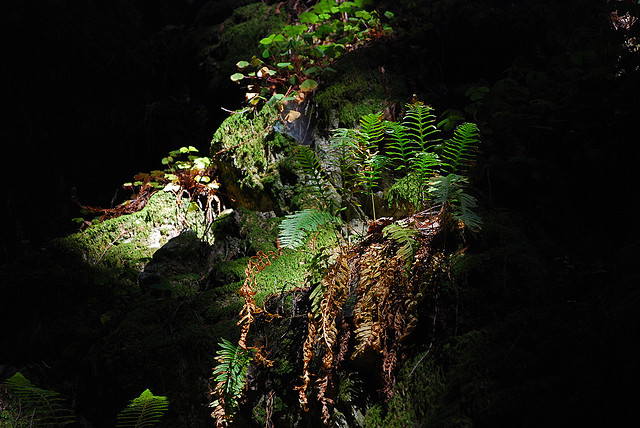The image depicts a dense section of vegetation, possibly within a forest or terrarium, illuminated by natural light amidst an otherwise dark setting. The scene is primarily centered, with an array of plant life extending from the top to the bottom of the image. The background is predominantly black, with the light illuminating the middle-left and middle sections, highlighting green, red, blue, orange, yellow, and black colors. Various leaves, some green and thriving, others brown and possibly drying, are visible. These leaves, along with moss-covered rocks, create a lush, tropical atmosphere. On the middle left side, moths rest on the rocks, blending into the plant life. The surrounding darkness and natural light evoke the feeling of being in a jungle or near a cave.